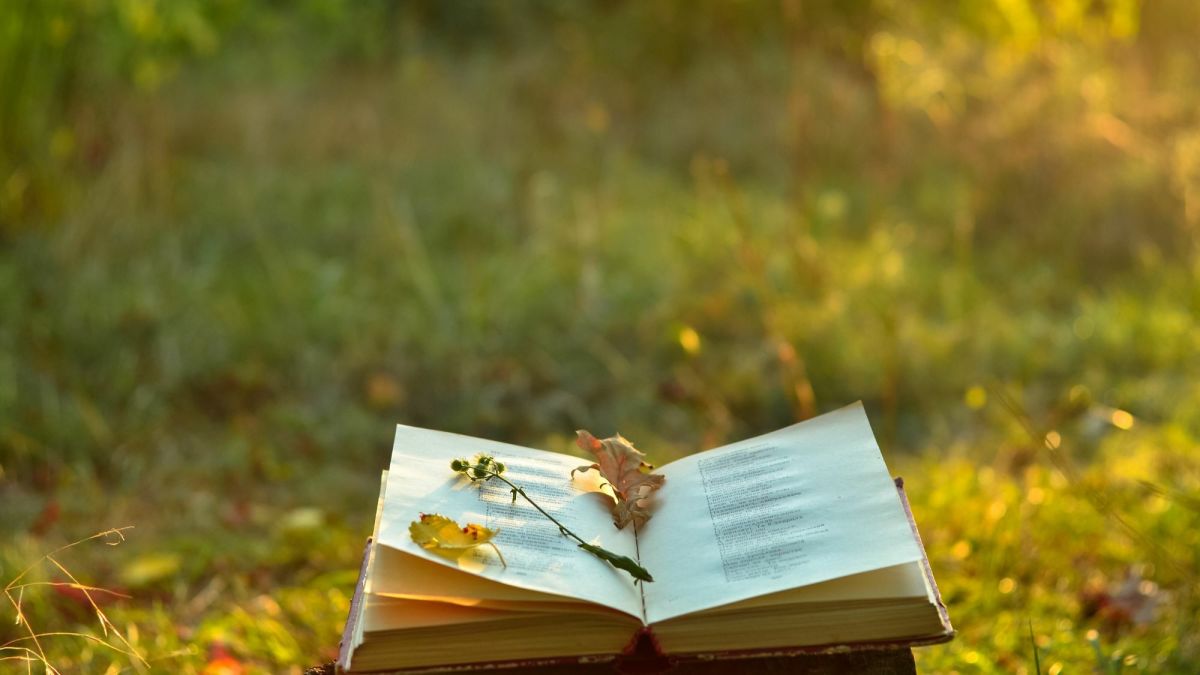This photograph depicts a picturesque, staged scene of an open book lying on the ground in what appears to be a grassy field or forested area, bathed in the golden light of a setting sun. The background, consisting of greens and earthy browns, is artistically blurred, suggesting tall grass, bushes, and possibly trees, typical of the end of summer or early fall. The book, likely a collection of poetry judging by the varied line lengths and stanza breaks visible on the slightly warped pages, is opened approximately halfway. Nestled within its pages is a delicate stem with small buds—possibly remnants of pulled-off petals—accompanied by two fallen leaves, one yellow and the other brown. Additional dry leaves are scattered around, enhancing the autumnal charm of the scene. The overall mood of the image is quiet and reflective, inviting the viewer to imagine the immersive experience of reading poetry amidst nature.